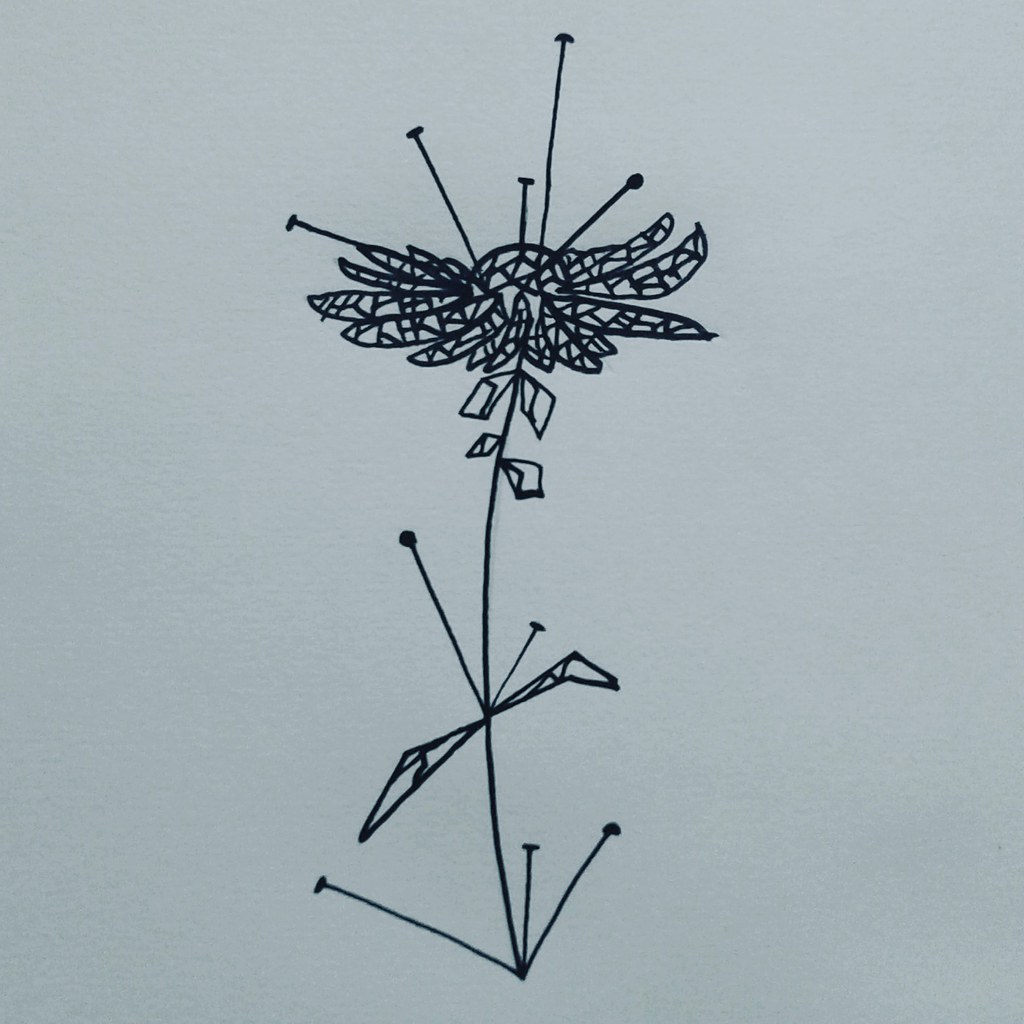This intricately detailed black ink drawing depicts a solitary flower set against a gray background. The flower features a delicate, slender stem that extends vertically, supporting a modest bloom at its apex. The petals are marked with intricate black lines, simulating natural creases and textures, and five stamens protrude prominently from the center. Below the flower, a few leaves attach to the stem, each intricately detailed with fine black lines. More leaves are positioned farther down the stem, accompanied by additional black lines that create an organic, naturalistic appearance. The petals appear as if they could be upside down, adding an element of curiosity and whimsy to the piece.